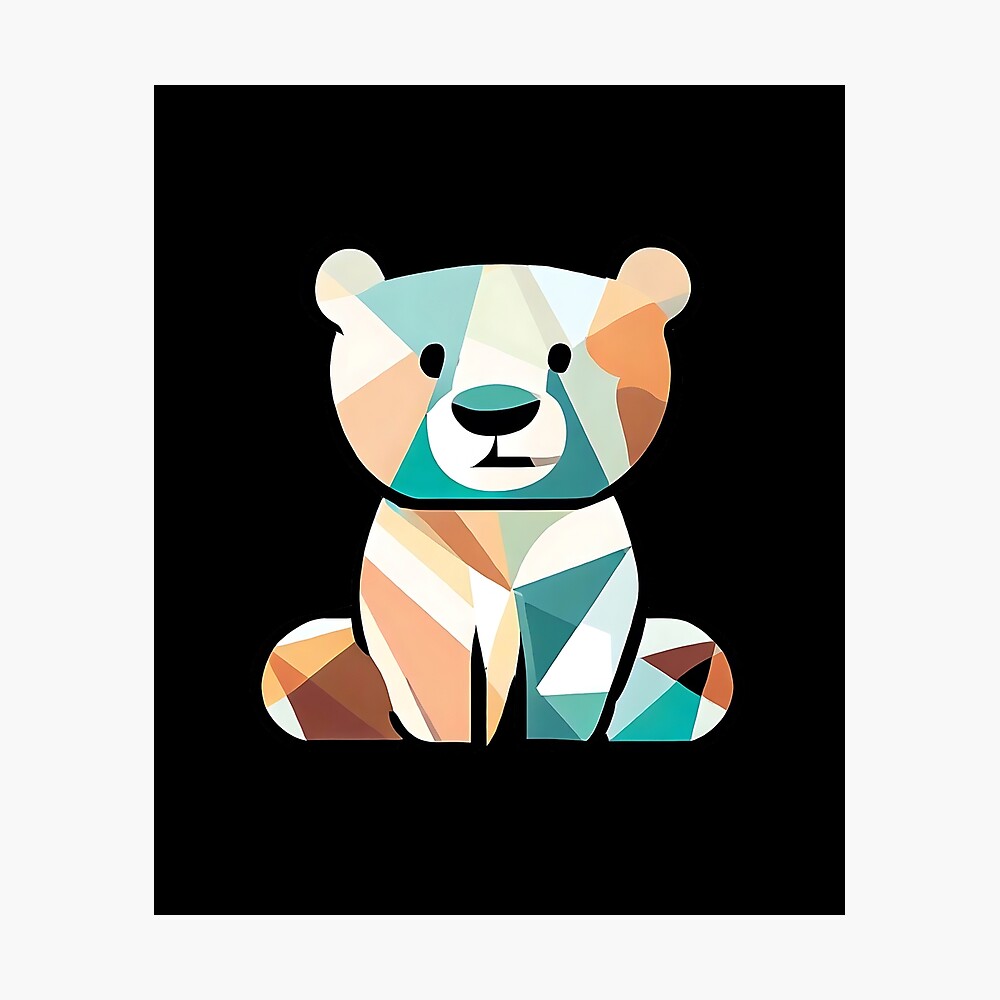The image showcases a digitally created depiction of a bear cub, characterized by its small and youthful appearance. The cub is seated with its paws in front and legs slightly spread, knees pointing outwards. The simplicity in the outline and design of the bear is contrasted by a vibrant and complex color palette, featuring an array of blues, oranges, greens, and both lighter and darker shades. The bear's gaze is directed straight at the viewer, adding to the overall charm of this colorful and aesthetically pleasing artistic rendition.